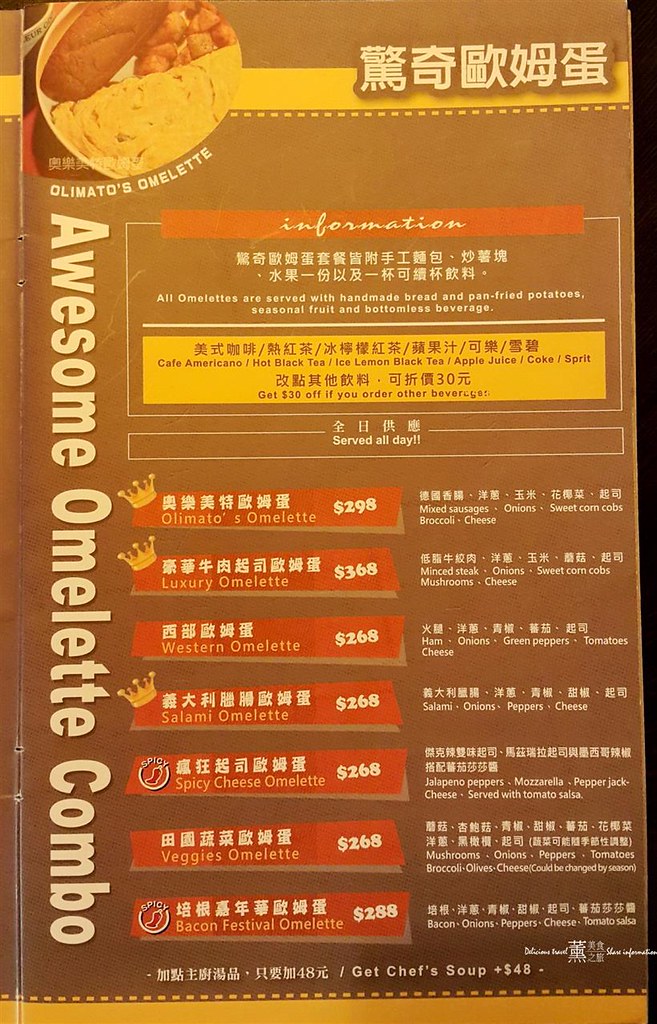**Captivating Menu Snapshot**

At the top of this photograph of a menu page, there's an enticing inset image featuring a delectable breakfast spread — eggs, crispy tater tots, and a slice of freshly toasted bread. The header proudly announces "Oli Motto's Omelette" with an "Awesome Omelette Combo" detailed in large, bold letters running down the left side.

Beneath a cursive "Information" header, a translated block of Chinese text reveals that all omelettes are served with handmade bread, pan-fried potatoes, seasonal fruit, and a bottomless beverage. The menu highlights the fact that these sumptuous breakfast offerings are available all day.

To quench your thirst, the beverage options include coffee, americano, hot black tea, iced lemon black tea, apple juice, Coke, or Sprite.

Below, the menu lists a variety of omelette selections, each accompanied by detailed descriptions of their unique ingredients:
- **Oli Motto's Omelette**
- **Luxury Omelette**
- **Western Omelette**
- **Salami Omelette**
- **Spicy Cheese Omelette**
- **Veggies Omelette**
- **Bacon Festival Omelette**

This menu presents a delightful array of options for omelette enthusiasts, each carefully crafted to cater to diverse tastes and preferences.